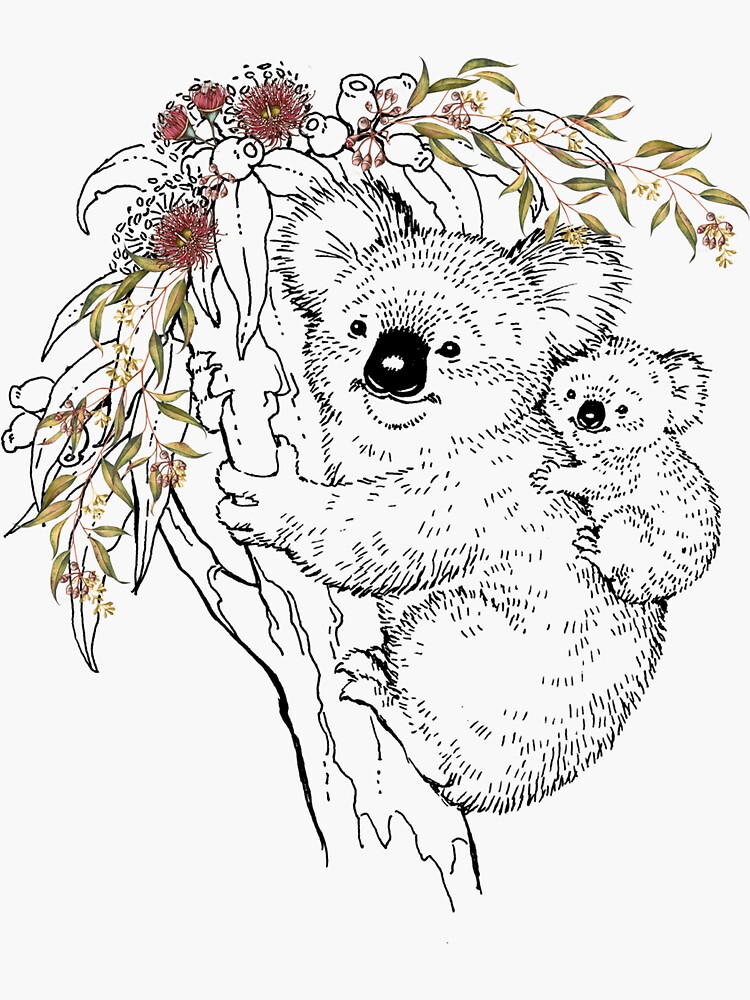This digital drawing features a heartwarming scene of two koalas – an adult and a child – resting on a tree. The child koala gleefully clings to the back of the adult, both appearing cheerful with smiles and expressive black eyes. The adult koala, likely the mother, holds onto the tree trunk with its claws. While the koalas and the tree trunk are rendered in black and white, offering a stark, illustrative contrast, the top of the tree is a burst of color. Green, teardrop-shaped leaves intermingle with vibrant flowers, including pinkish-red bellflowers and line-adorned blooms, adding a splash of life to the drawing. The details like the koalas' fluffy ears, black noses, and the intricate floral elements make this image both charming and detailed, resembling a potential coloring sheet.